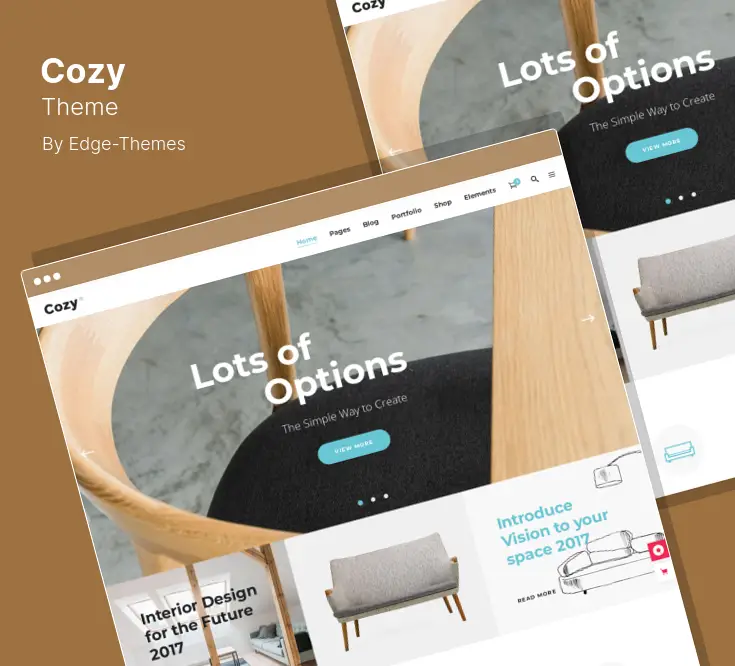This promotional graphic for the Cozy theme by EdgeThemes highlights its versatility, underscored by the tagline "Lots of Options," emphasizing the theme's simplicity in website creation. The centerpiece of the graphic is a large screenshot of a website utilizing the Cozy theme, showcasing its modern and minimalistic design elements. The website features a prominent header image with overlay text and a "View More" button, directing users to further content.

The website preview includes sections dedicated to interior design, with headlines such as "Interior Design for the Future 2017" and "Introduce Your Vision into Space 2017," accompanied by images of stylish furniture like chairs and sofas. The navigation menu at the top displays options for Home, Pages, Blog, Portfolio, Shop, and includes icons for search and account functionalities, ensuring a comprehensive browsing experience.

The background of the promotional graphic is a warm brown hue that enhances the cozy aesthetic, making the theme's name quite apt. This color choice enriches the overall inviting and comfortable feel that the Cozy theme aims to deliver.